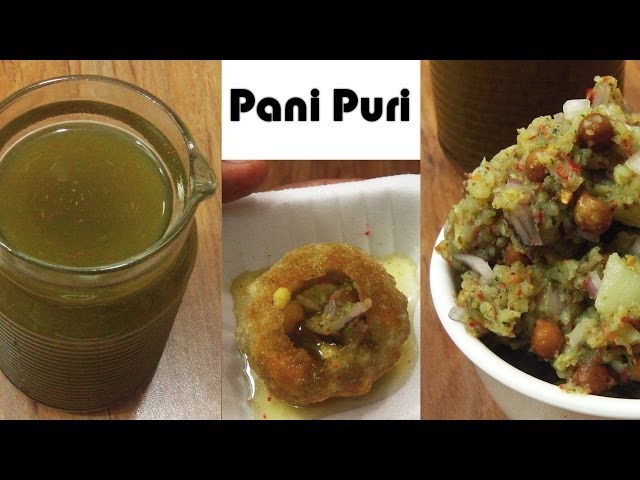The image is a composite of three distinct photos, set against a consistent wooden background and bordered in black on the top and bottom. On the left, there's a clear glass jar with a spout, filled with a green, grayish liquid that contains swirls of orange and creamy white herbs or seeds. This jar is placed on what appears to be a wooden table. The central photo features a white styrofoam tray holding a round, fried food item—likely a piece of Pani Puri—filled with various ingredients and surrounded by a small puddle of liquid. Above this item, a white box with black text spells out "Pani Puri." A thumb is visible at the top, holding the tray securely. The rightmost photo shows a white bowl containing a herbed mixture of rice, brown chickpeas, and slices of onion, also displayed on a wooden surface. The jar from the left side is partially visible in the background of this photo. This triptych may serve as an advertisement for a YouTube video, blog, or website.